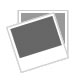This detailed photograph captures an aged, small wooden Easter basket filled with artificial Easter grass and three colorful, synthetic chicks. The basket, which has a handle and appears quite old, is sitting on a green, old-fashioned glass plate. The three chicks inside boast bold, non-natural hues: one hot pink, another dark green, and the last a mix of light green, yellow, and white. The glass plate beneath the basket exudes a vintage charm, possibly made of a stained or milk glass type. This setup is positioned on a table adorned with a tablecloth that features a cream-colored base and green patterned lines, giving it an older, nostalgic feel. The background includes a hint of another cloth with a white and blue floral pattern, suggesting a cozy, possibly picnic-like setting.